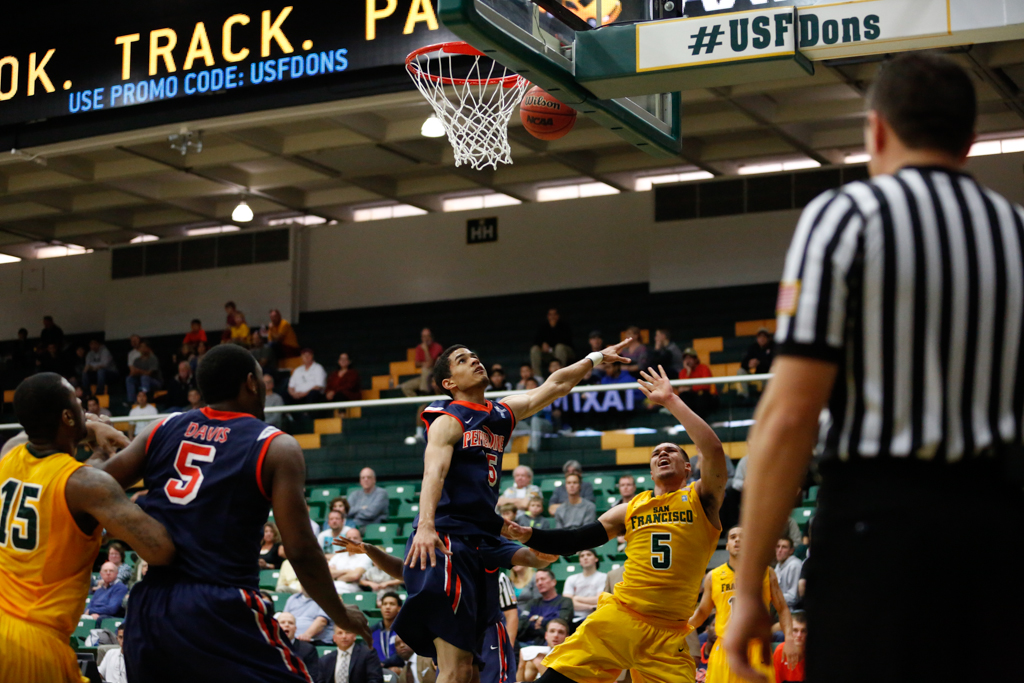In this dynamic photograph of a basketball game between the San Francisco Dons and Purdue, the intense action centers around a player with light brown skin and dark hair, clad in a navy blue uniform with red accents, sponsored by Nike. He’s intently looking up at the basket, poised to see if his shot will go in, although the ball, emblazoned with "Wilson" and "NCAA," appears to be too low to make it. Flanking him on his left is a teammate with dark skin, also in navy blue, while an opponent in a yellow and green uniform vies for position. To his right stands another light-skinned adversary in yellow. A referee, slightly blurred, in classic black and white stripes, supervises the action from the left foreground. Towering above them, green and yellow stands, though only about a quarter full, host an engaged crowd. At the top of the image, promotional banners and the code "USFDONS" hint at a special offer, adding a commercial touch to the scene.